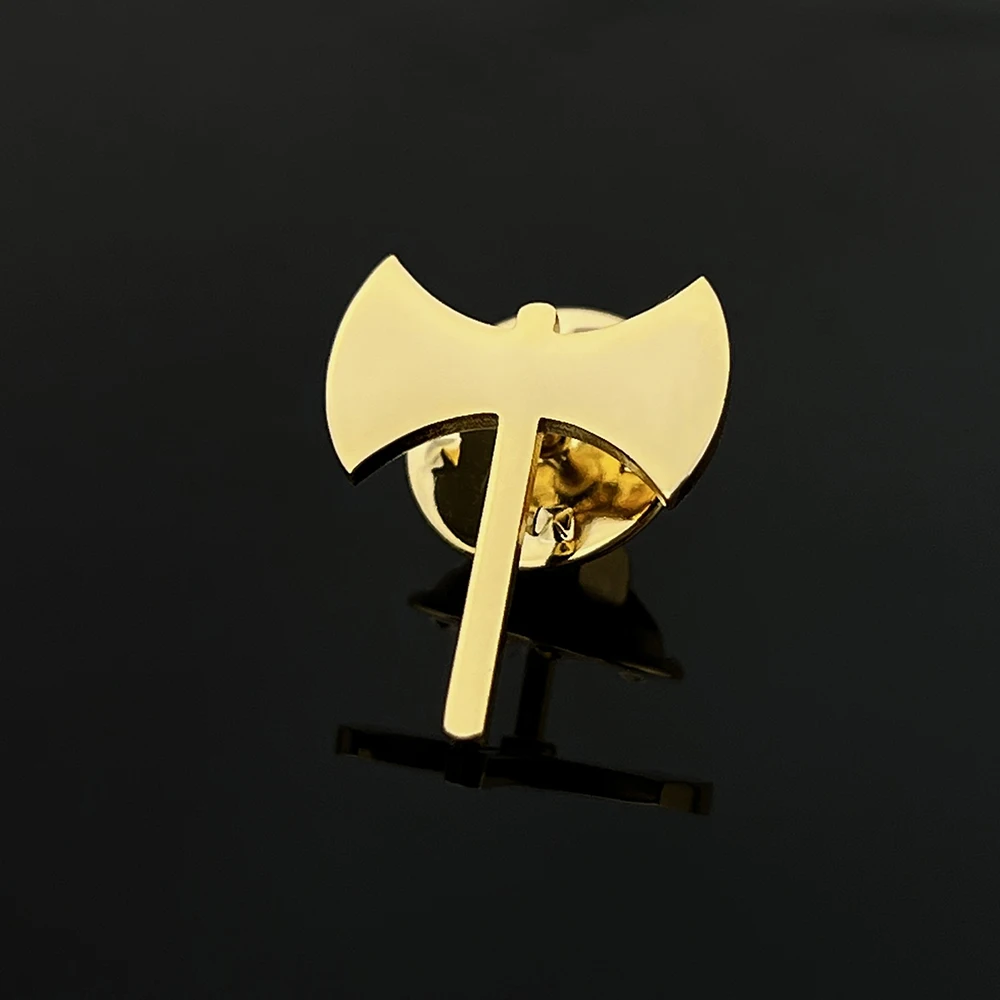Set against a flat, all-black background, the image prominently features a highly detailed, gold-colored double-sided battleaxe. The battleaxe, possibly a cufflink or an earring given its reflective, close-up appearance, hovers slightly rotated above a deep yellow circular disk. The axe itself is devoid of any markings and shines with a uniform gold luster, while its handle is notably twice as long as its blades. Below the axe and disk, their reflections can be seen subtly mirrored against the dark surface, adding depth to the composition. The scene is devoid of people or additional text, focusing entirely on the gleaming, intricate details of the battleaxe and its accompanying disk.